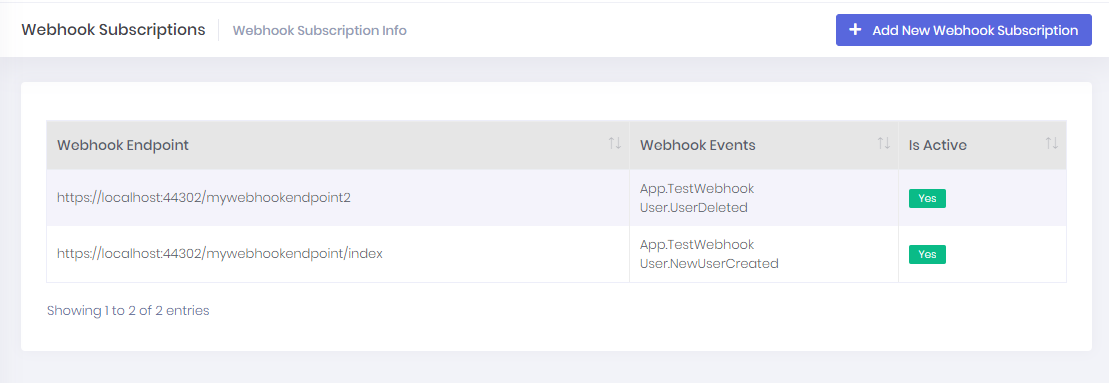The top left corner of the image displays the "Webhook Subscriptions" section. Within this section, there is a blue rectangular button featuring a plus sign and the label "Add New Webhook Subscription." Adjacent to this button is a gray area containing a button labeled "Webhook Endpoint." Below this, the status "Webhook Events is Active" is indicated, accompanied by the text "https://localhost:44302/mywebhookendpoint2."

Further down, an entry titled "testwebhookuseruserdeleted" is listed, followed by a gray square with the text "Yes." This same URL, "https://localhost:44302/mywebhookendpoint2," is displayed again. The view shows one or two entries, indicating that there might be a variation in the number of displayed items.

The topmost row of the section is shaded in gray, transitioning from dark gray, to light gray, and then to white. Arrows are also present in this white area, suggesting navigational icons or sorting functionalities.